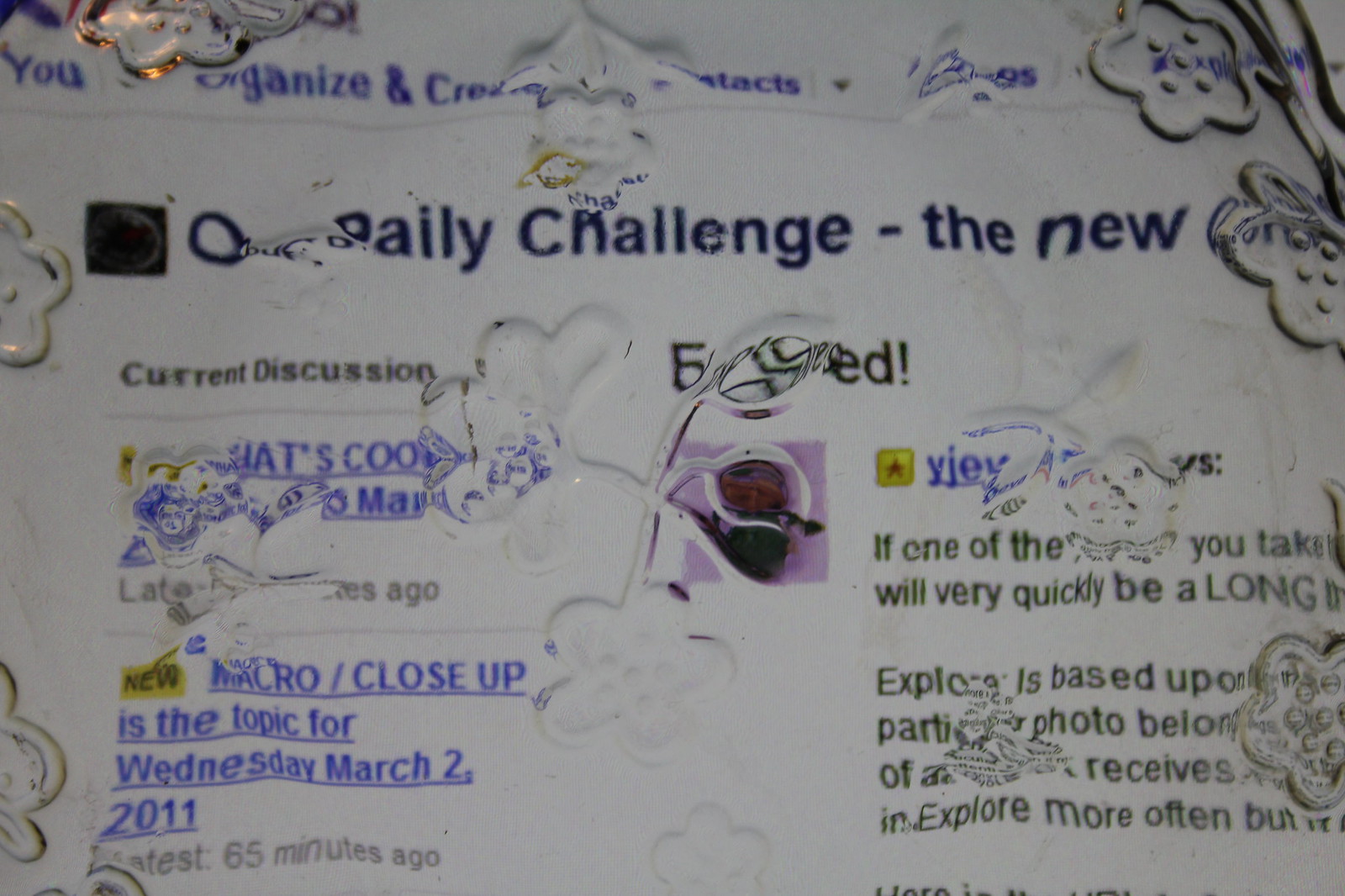The image depicts a white paper-like card that seems to have been altered or distressed, giving it a fabric-like appearance with water splashes and possibly glued or sewn-on elements such as buttons and flowers, which distort the text. The card's main heading at the top reads "Daily Challenge." In various sections, there are purple and blue words interspersed with black text and blue splotches. The text towards the bottom references a topic for Wednesday, March 2nd, 2011, identified as "Macro/Close-Up." 

The layered elements, such as flowers that blur parts of the card, make deciphering the text challenging. However, phrases like "You organize and create" and "Daily Challenge" are distinguishable, and there are mentions of “current discussion” and "latest 65 minutes ago." The right side of the card includes fragments of words like "explore" and what might be "contact" or "contexts." The overall design suggests an interactive format that one might find on a website, with distorted clickable elements and decorative overlays.